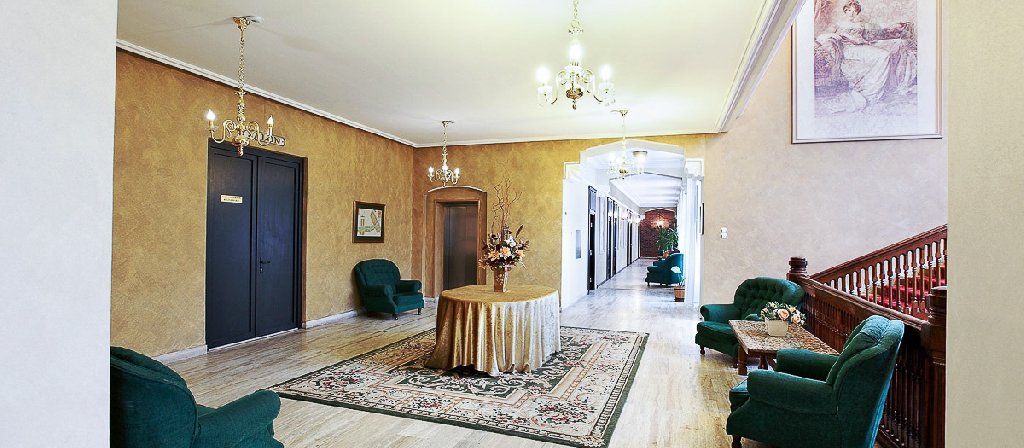This image depicts a luxurious common area or lobby, potentially of an older, elegant hotel or office building. The foreground features four velvet green armchairs, each positioned in a corner of the room. Central to this space is a Persian-style rug beneath a large, round table adorned with a gold tablecloth and a vibrant flower arrangement. A grand chandelier hangs in the center of the room, complemented by two smaller chandeliers on the left side.

On the left-hand wall, two doors are visible beneath a picture, while another portrait, likely of a woman from a bygone era, hangs adjacent to a brown staircase that ascends to another level. This staircase is located on the right side.

The background reveals a long hallway lined with additional chairs and multiple doors along the left-hand side, suggesting the possibility of hotel rooms or offices. The overall ambiance indicates a space designed for both comfort and opulence.